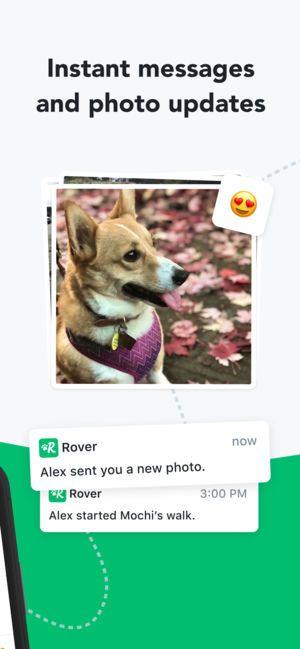The image features a text banner at the top, centrally aligned in black font on a grey background, that reads "Instant Message and Photo Update." Below this, there is a stack of photos, with the topmost one prominently displayed. This visible photo showcases a dog with its tongue out, wearing a brown collar with a yellow tag and a brown emblem, as well as a purple vest adorned with some lines. A yellow emoji with red heart-shaped eyes is positioned at the top-right corner of the photo, indicating a live update.

Beneath the dog's photo, there are two text notifications. The first notification reads, "Rova: Alex sent you a new photo," and immediately below it is another notification stating, "Rova: Alex started Mochi's walk. 3:00 PM." Both notifications feature an icon next to the name "Rova," which is a white letter "R" coupled with a paw print on a green background. The lower part of the image also has a green background, providing a cohesive look to the overall design.